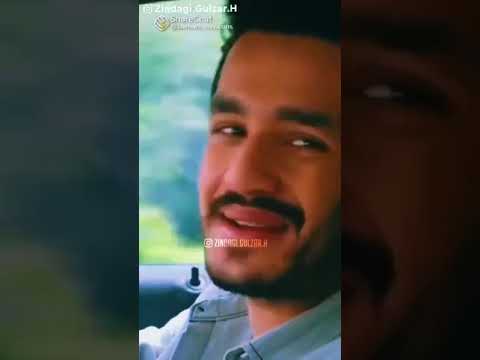The image is a rectangular photograph that is slightly wider than it is tall, displaying the close-up face of a man in the center. This main image is superimposed over a blurred, darker background of the same scene, leaving only the central photo clear and detailed. The man appears to be in his late 20s to early 30s, has light brown skin, a short black beard and mustache that do not cover under his lips, and dark brown eyes. He has black hair and is smiling towards the right side of the image, with his eyes slightly angled in that direction as well. He is wearing a light blue collared shirt that is unbuttoned at the top, possibly a denim long-sleeved button-down shirt. Behind him, there is a verdant, blurry scenery visible through what seems to be a car window, with a black area and a vertical cylinder resembling a window button indicating he's inside a vehicle with a black vinyl interior. There are also discernible white or gray words and a watermark in the top left corner reading "Zingdagi Gulzar dot H" with an additional logo beneath it, as well as another watermark in the center of the image.